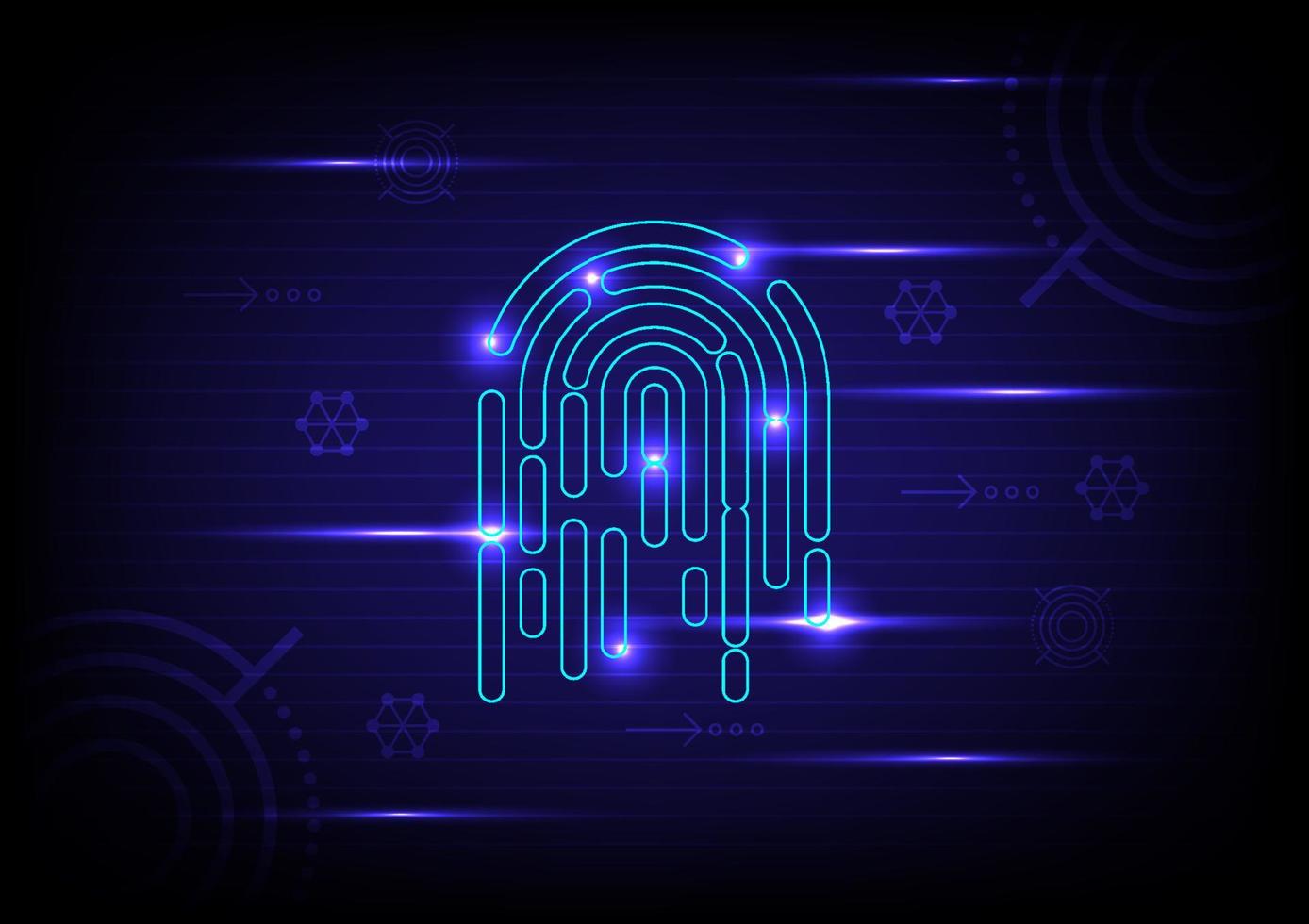The image is a high-tech, computer-generated abstract art piece with a vibrant, dynamic design. The central area features a unique, maze-like pattern made of segmented and rounded sections that almost resemble a cylindrical shape composed of pill-like segments. This central figure is bathed in bright, turquoise light with purple highlights, creating an impression of movement and life. Surrounding this main structure, there are eight smaller abstract images, likely hexagonal or circular, interconnected by bright blue, pink, and purplish lights. These lights stretch horizontally across the background, enhancing the overall futuristic feel. The background itself is a rich blend of purple and black, accented by metallic, circular, and hexagonal designs. At the bottom corners, heliocentric circular objects chain together, focusing attention towards the illuminated center. This black outer gradient further intensifies the vibrant colors and lights emanating from the center, giving the entire image a neon-lit, almost alive appearance.